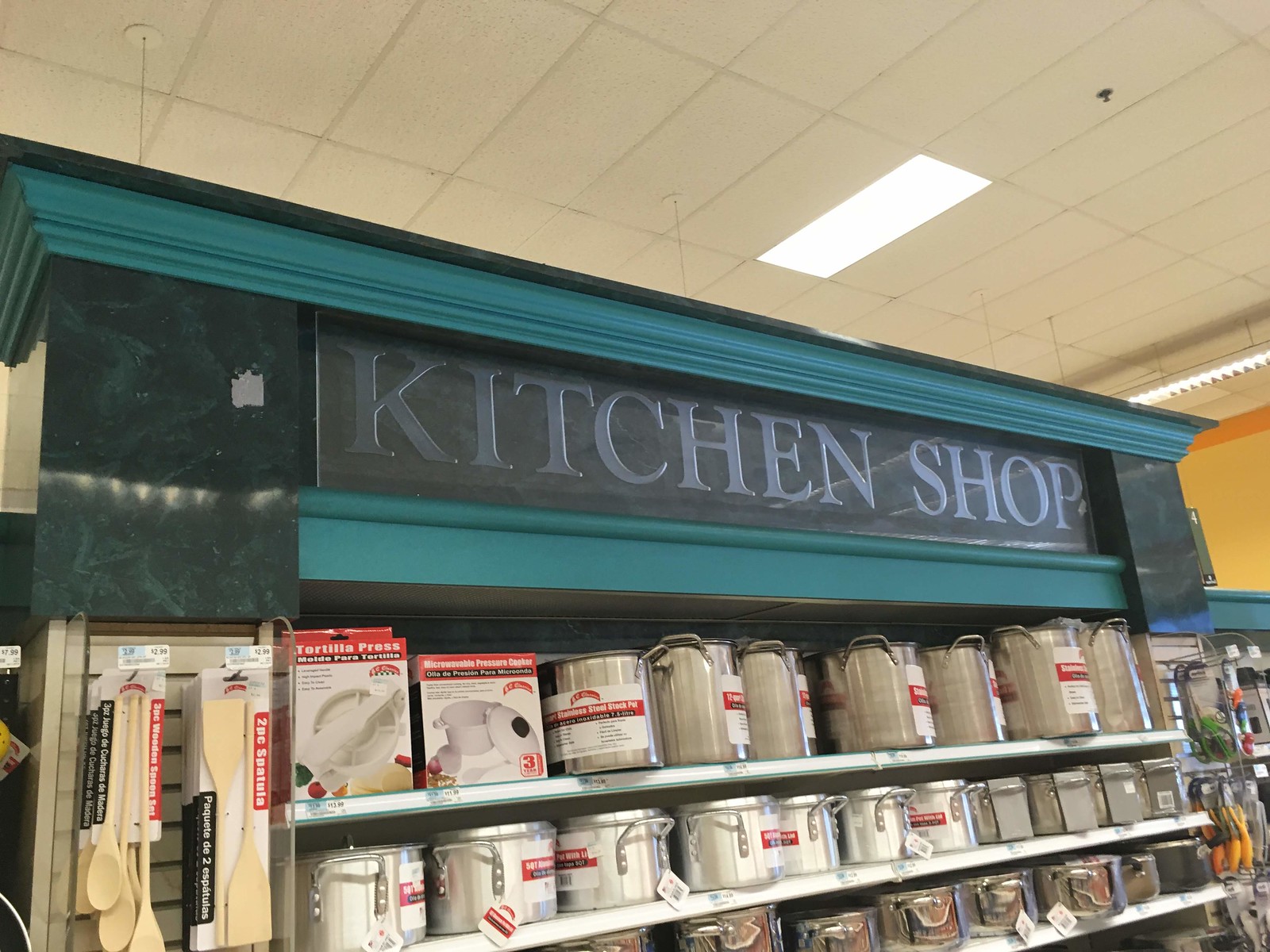**Detailed Caption:**

The image showcases the interior of a store, specifically focusing on a display shelf. The vantage point is slightly from the left. At the top of the display, the words "Kitchen Shop" are prominently displayed in a grayish-blue font against a gray background. The shelving units are blue, with tapered tops and bottoms, offering a sleek and modern aesthetic. The edges of the display are accentuated with greenish-teal granite, adding a touch of sophistication. 

The central part of the display is filled with large, silver, and shiny metal pots. Each pot has a white label attached to it along with a small red tag. The labels feature black writing, although the specific text is not visible. Adjacent to this, on the left edge of the display, there is an arrangement of wooden utensils hanging from hooks. The utensils include wooden spatulas and spoons, mounted on white cards with a black edge. A red indicator, written vertically, is part of these cards, although the text is not legible. 

To the right, more kitchen utensils and accessories can be seen hanging, contributing to the well-organized and comprehensive layout of the Kitchen Shop display.